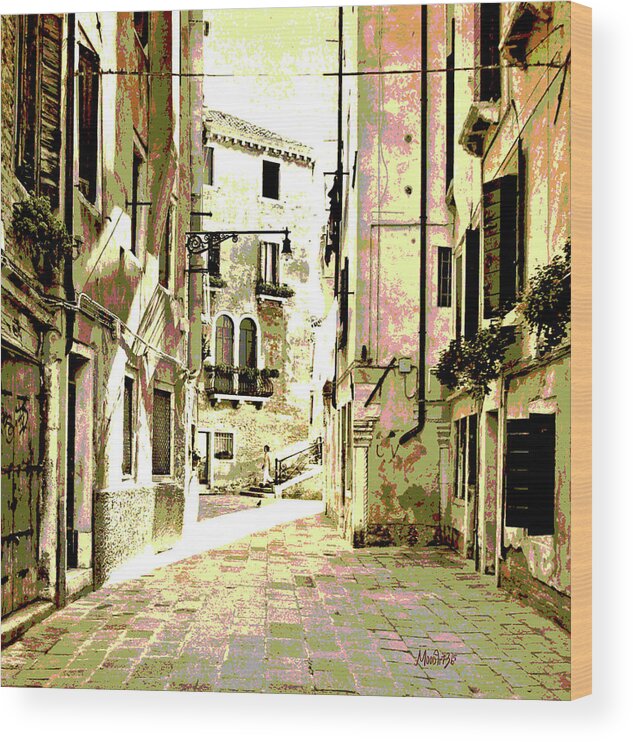This image depicts a narrow European alleyway, possibly in a village or small town, with a distinctive green and pink pastel color palette. The street is paved with cobblestones and framed by three to four-story buildings featuring a mix of rounded and square windows, some adorned with shutters and flower boxes. The left side of the alleyway is characterized by darker green and pink hues while the right side showcases lighter green tones and pale orange accents. Various plants spill from window boxes and balconies, and an iron bar with a hanging light extends from a building on the left. Near the center of the image, a woman in a white dress is walking down a staircase towards the cobblestone path. The overall look is heavily edited or artistically rendered, giving it a slightly washed-out, vintage appearance. A stylized, barely legible signature that begins with the letter 'M' appears in the bottom left-hand corner, suggesting it might be an art print or a painting. The scene is marked by an old-world charm, reflecting the architecture and ambiance of a bygone era.